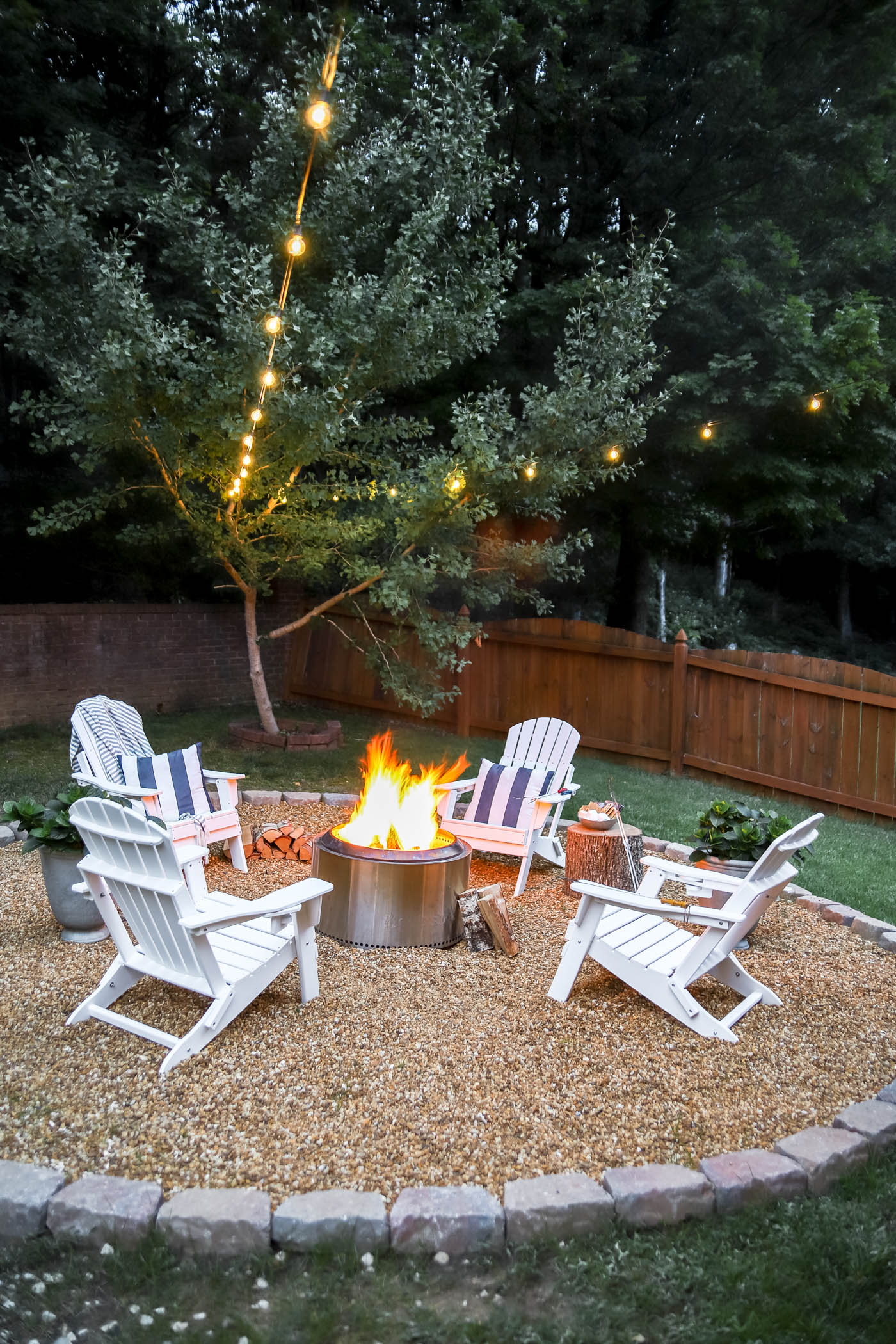This portrait layout photograph captures an inviting outdoor yard setup, positioned on a lush green lawn. At the center of the image is a circular stone structure filled with tiny orange and white gravel. Enclosed within this circle, a prominent metal fire pit with vibrant orange and yellow flames takes center stage, surrounded by four white Adirondack chairs. Two of these chairs, positioned farthest from the fire pit, are adorned with blue and white striped pillows, while one also drapes a matching towel over its back. Between some of the chairs, vibrant potted plants add a touch of greenery. Overhead, two strings of glowing yellow lights are strung from a tree towards the camera, creating a cozy ambiance. The background features a horizontal brown wooden fence running through its center, with towering trees and rich foliage adding a serene, natural backdrop to the scene. The bottom part of the image transitions from gravel to green grass, with small white rocks speckled towards the left.